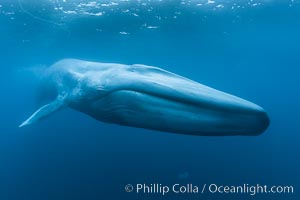This captivating underwater photograph, taken by a professional photographer and credited to philipcolla.com, features a humpback whale swimming just below the ocean surface. The image is predominantly blue, with lighter shades created by sunlight filtering through the water, casting a serene yet striking contrast against the darker ocean depths. The whale, discernible with its characteristically narrow head, long mouth, tiny eye, and identifiable fins, is positioned centrally and occupies most of the frame, emphasizing its immense size. Although the whale's entire body is not visible, the section from its mouth to the area past its fins is clearly defined, showcasing its streamlined form as it descends gracefully through the water.